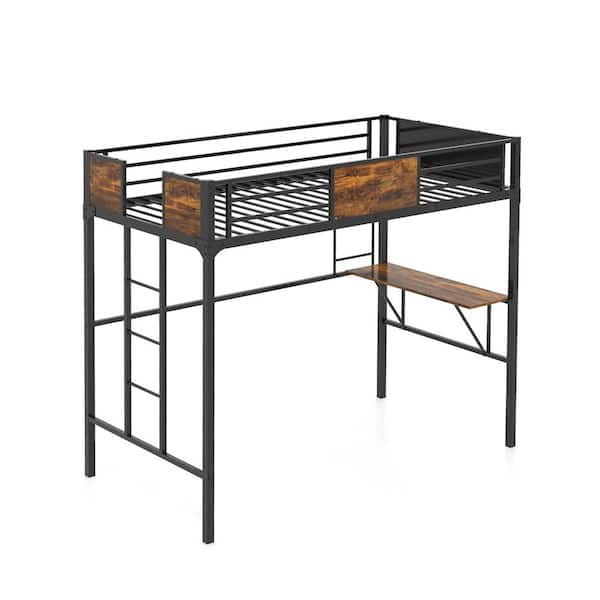This photograph captures a uniquely designed metal shelf or rack, viewed diagonally. The structure features four legs providing a sturdy base. On the left side, there is a small, three-step ladder that leads up to the top. The top surface is not solid but made of a metal grating, encased with a railing that includes built-in wooden panels, adding an artistic touch. Stretching across the length of the shelf are supportive bars, ensuring stability. Just beneath the main shelf on the right side, there is a smaller wooden shelf. Artistic wooden elements are integrated throughout the design, enhancing its aesthetic appeal without contributing to functionality. The majority of the rack is black, blending industrial and artistic influences in its overall appearance.